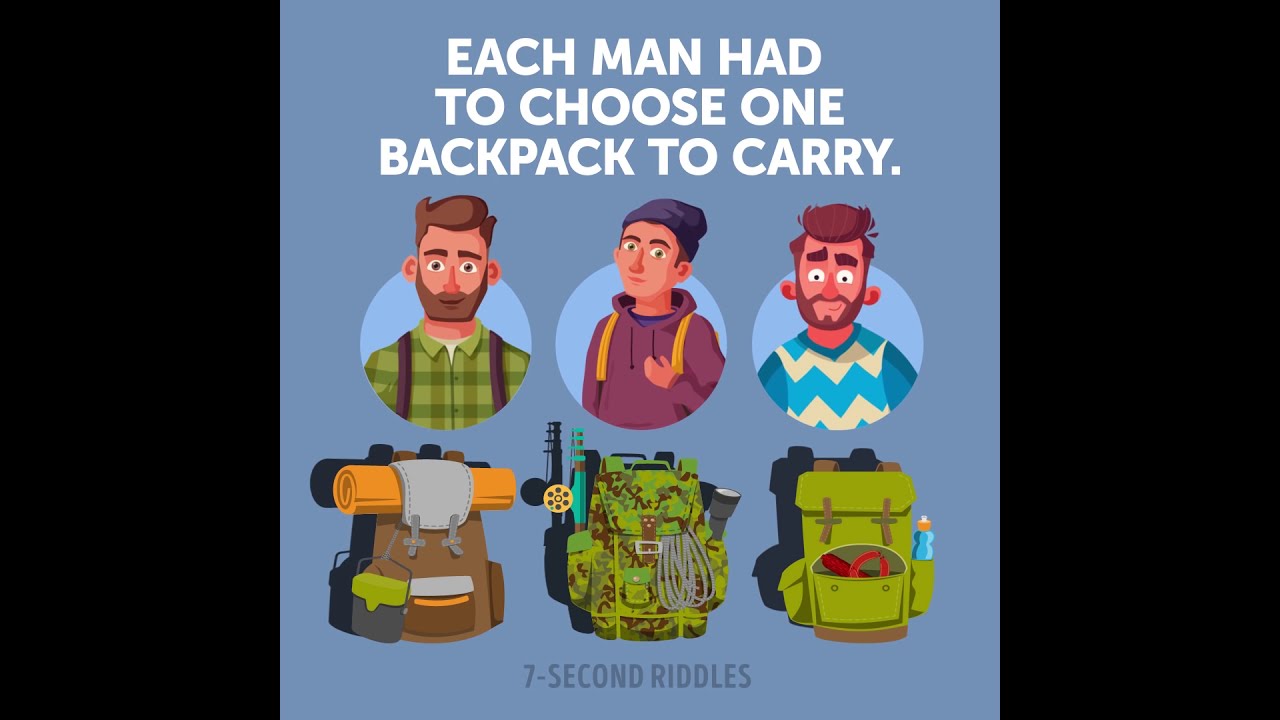This image is a detailed color illustration set within a rectangular frame with black bars on the far left and right, focusing attention on the central square picture. The background is a periwinkle blue. At the top, in white uppercase block lettering, it reads: "EACH MAN HAD TO CHOOSE ONE BACKPACK TO CARRY." Below this text, three cartoon characters are depicted from the bust up, each set within light blue circles.

On the far left is a character resembling a lumberjack, a Caucasian man with fair skin, green eyes, brown wavy shortcut hair, and a full beard. He is wearing a green plaid shirt with brown suspenders. 

In the center is a young boy of Caucasian descent, sporting a blue-purple beanie and a purplish-red hoodie, with yellow backpack straps over his shoulders.

On the far right is a man with unruly brown hair, thick eyebrows, and a beard. His ears stick out noticeably. He is wearing a blue and white chevron-patterned sweater vest and has a lighthearted, smiling expression.

Directly below each character is a corresponding backpack. The backpack on the far left is brown with an attached gold bedroll on top and a green-topped black container hanging from it. The center backpack features a green army camouflage design with various implements sticking out, including a blue fishing rod, a black flashlight, and some rope. The backpack on the far right is a simpler design in green, with a fold-over top, some red objects in the pouch, and a blue water bottle attached to the right-hand side.

At the bottom center of the illustration, in light gray text, it says "SEVEN-SECOND RIDDLES."